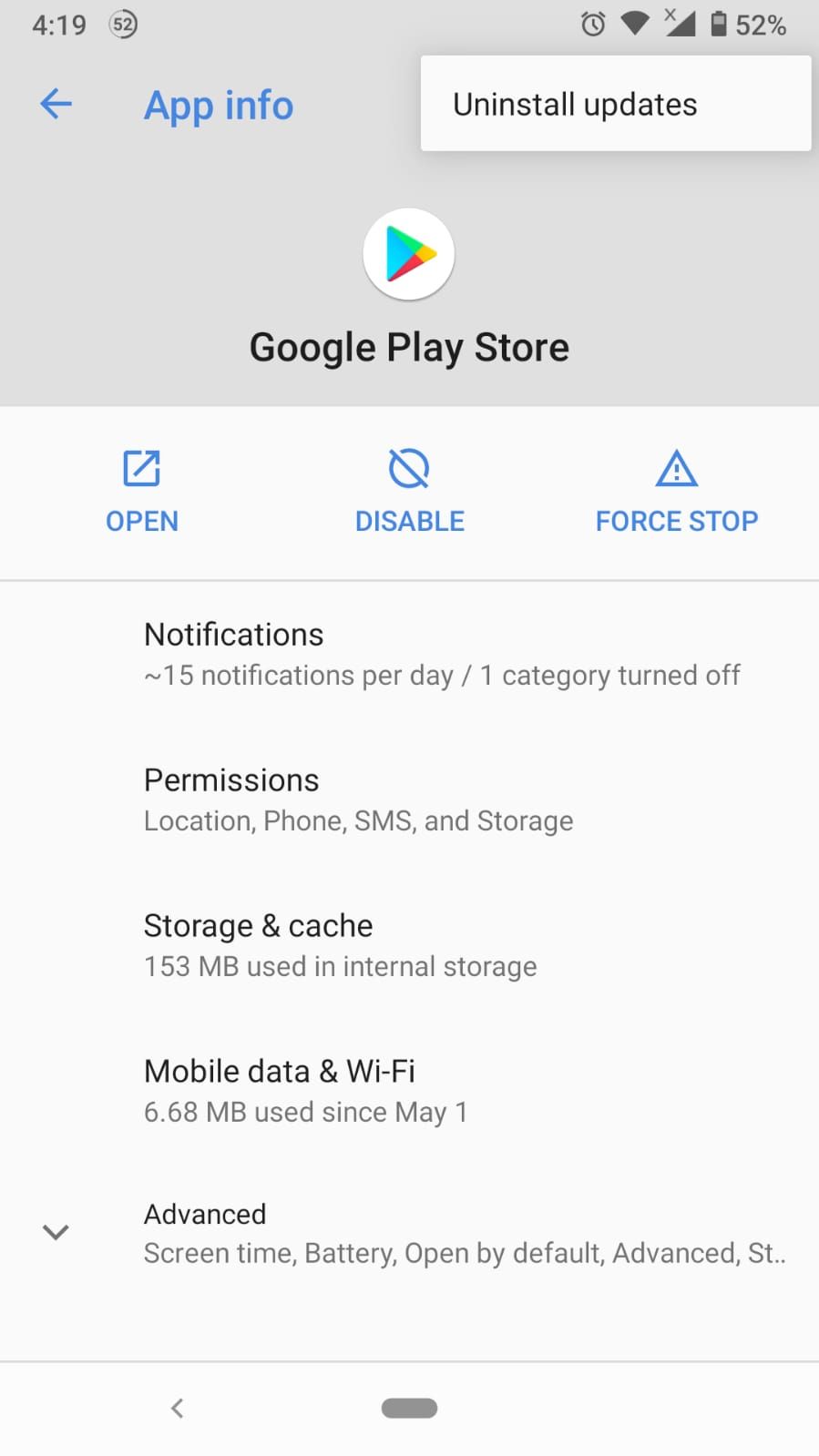In this image, we see a screenshot from an Android phone displaying the "App Info" page for the Google Play Store app. At the very top, there is a leftward-facing arrow for navigating back, and an option to uninstall updates located in the top right corner.

Below the title "App Info," several command buttons are visible. These include "Open," "Disable," and "Force Stop." Further down, detailed information about the app is presented:

- **Notifications:** This section indicates that the app sends 15 notifications per day, with one notification category turned off.
- **Permissions:** The app has access to Location, Phone, SMS, and Storage.
- **Storage and Cache:** The app uses 153 megabytes of internal storage.
- **Mobile Data & Wi-Fi:** The app has used 6.68 megabytes of data since May 1st.
- **Advanced:** This section includes additional settings such as Screen Time, Battery usage, Open by Default, and more, although the last option is partially cut off.

This comprehensive view provides a clear summary of the app's settings and usage statistics.